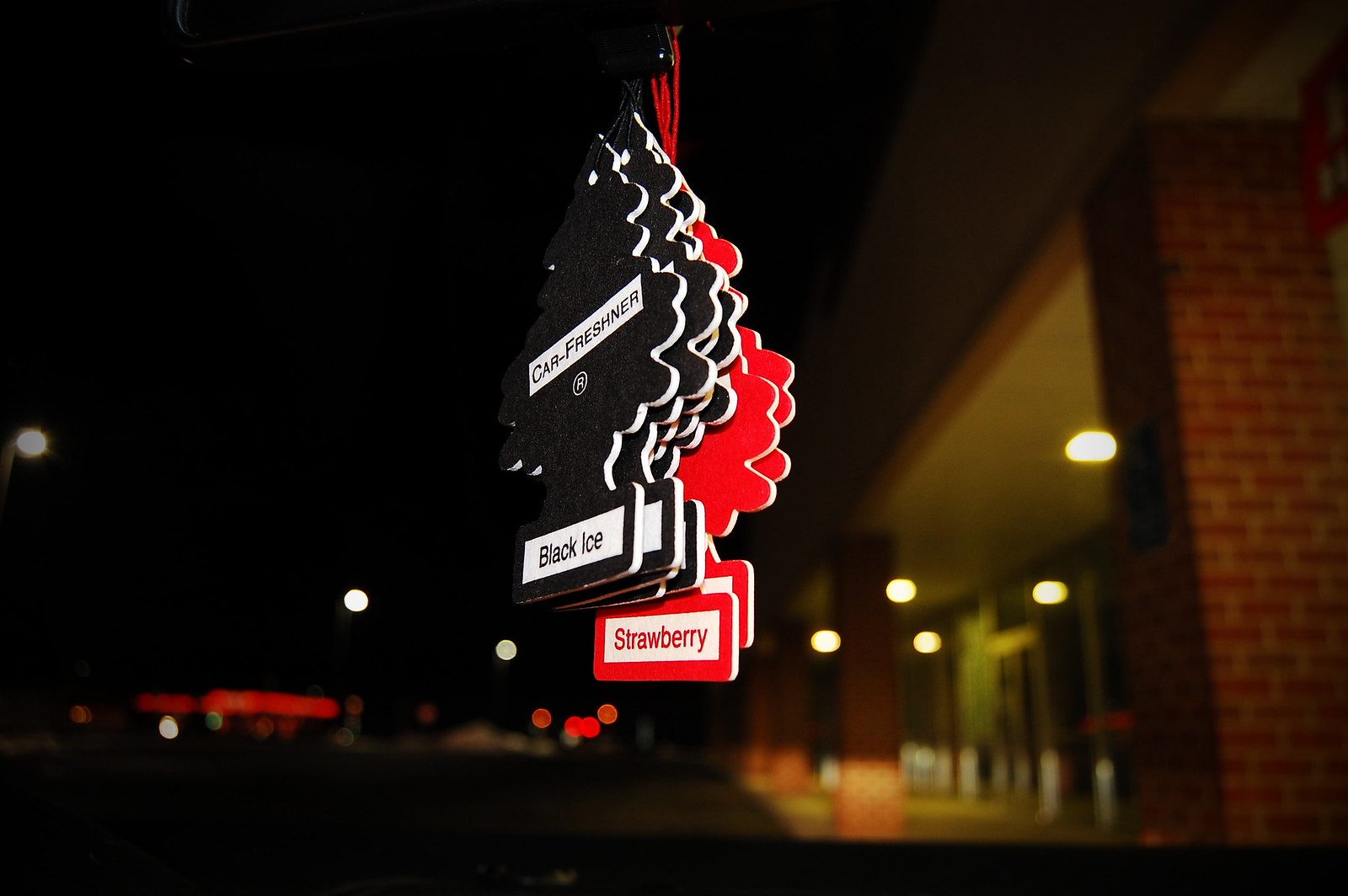The photograph captures a night scene, predominantly dark, with the focal point being a cluster of car fresheners of the tree variety. These air fresheners, five black and two red, are hanging from an indiscernible object, likely inside a car since an interior light makes them stand out vividly against the dim background. The black ones prominently display two white stickers, with "car freshener" on the upper sticker and "black ice" on the lower. Similarly, the red fresheners have white stickers at the bottom reading "strawberry" in red lettering. The backdrop reveals the night sky with a few street lights and faint images of buildings; to the right, there's a distinctly visible brick building that appears to be part of a plaza. The left side shows blurry, illuminated structures possibly belonging to a distant gas station or another building, casting a subtle glow to the otherwise shadowed setting.